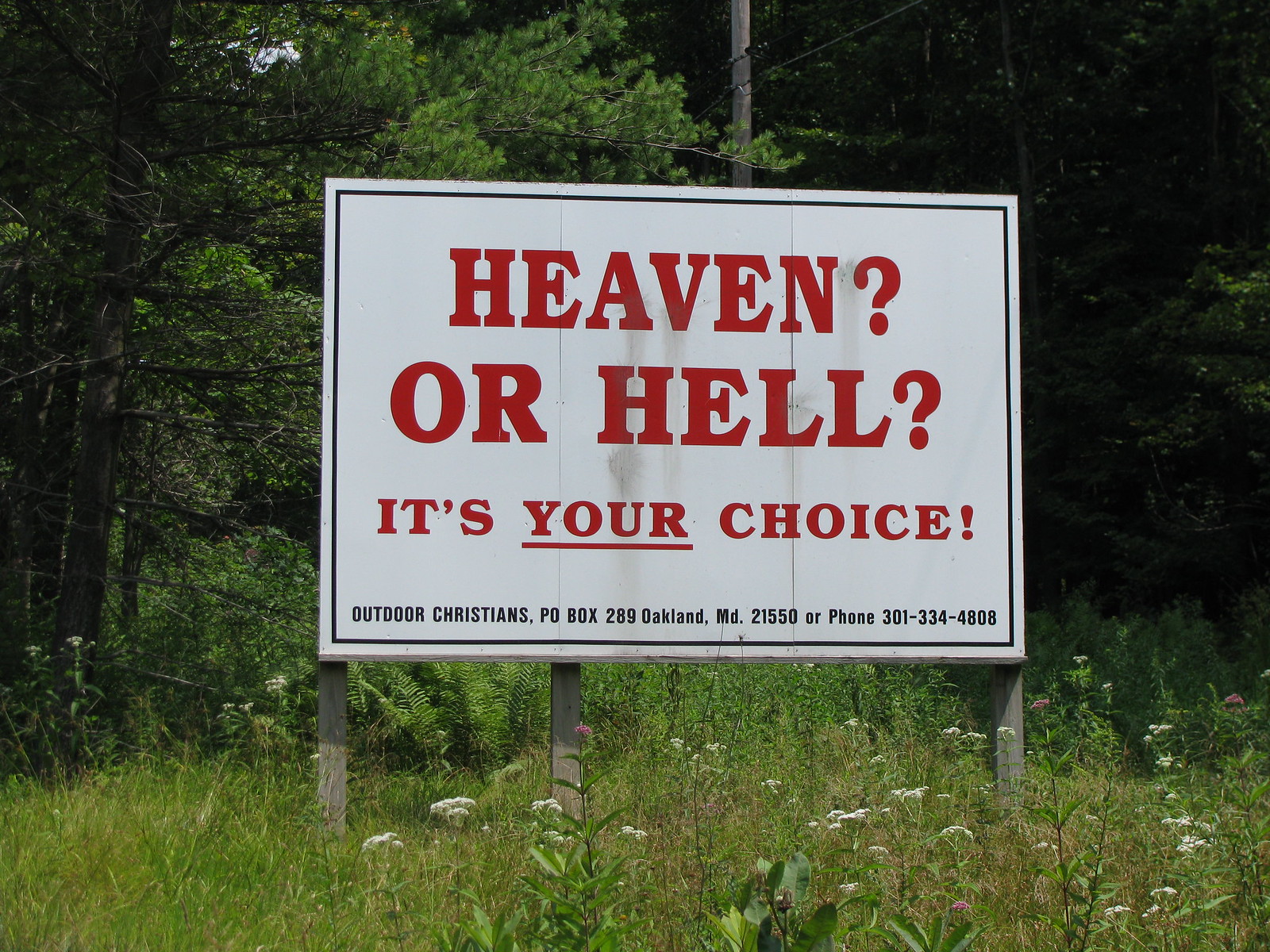The photo features an aged sign staked into the ground amidst a field overrun with wildflowers and weeds. The sign, which has a thin black border, is prominently white with red text that reads, "Heaven? or Hell? It's YOUR choice!" where "YOUR" is underlined and emphasized with an exclamation mark. This message invites contemplation of one's eternal destiny. At the bottom of the sign, finer print provides contact details: "Outdoor Christians, P.O. Box 269, Oakland, Maryland 21550, Phone: 301-334-4808." In the background, a shaded treeline marks the edge of the field, suggesting a cooler, serene forested area beyond the sign's stark warning. The weathered condition of the sign, marked by spots and signs of age, indicates it has been there for some time, heralding its message to passersby.